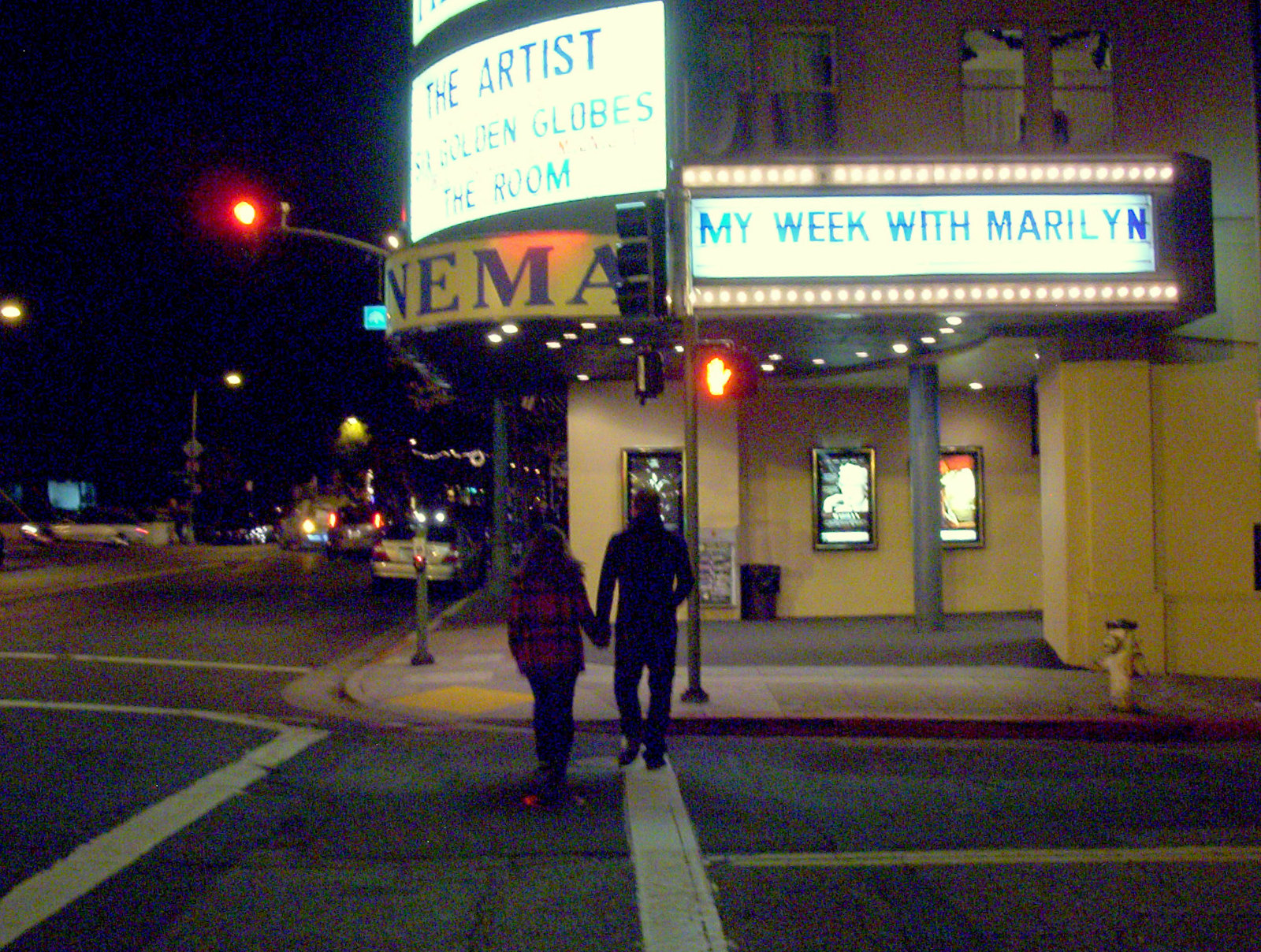A photograph taken at night captures a couple crossing a city street at a crosswalk. The man, dressed in a black jacket and black pants, walks on the right side of the crosswalk, holding hands with a woman in a red and black plaid lumberjack jacket. Her hair falls over her shoulders as they walk just in front of a cinema illuminated by marquee lights. The cinema’s marquee displays the titles "My Week with Marilyn," "The Artist," "Golden Globes," and "The Room" in blue letters against a white background. The marquee, outlined with light bulbs, casts a glow on the otherwise quiet street. Above the marquee, there are windows with curtains, suggesting residential spaces above the cinema. There are movie posters on the theater wall and a trash can to the left of the posters. Further framing the scene, a fire hydrant and a street lamp are visible on the right. The curb is painted red and includes a wheelchair-access drop-down in front of the theater. A white car is parked around the corner, and few other cars are visible in the distance. The overall atmosphere is calm, capturing a tranquil moment in a bustling city at night.